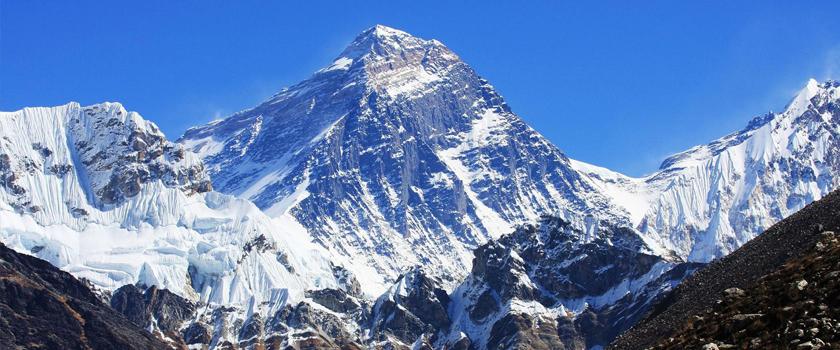The image features a stunning panoramic view of a mountain range dominated by three prominent, snow-capped peaks that occupy approximately 85 percent of the frame. The central peak, the tallest and most imposing, has less snow compared to the thick, snow-laden peaks flanking it on either side. The entire scene is bathed in crisp detail, emphasizing the substantial snowfall on the left peak, especially thick beneath it, and the contrasting rocky terrain visible at the corners of the frame, free of snow. The foreground consists of dirt piles suggesting proximity to the camera, adding depth to the high-definition photograph. A vibrant blue, cloudless sky stretches behind the mountains, emphasizing their grandeur and perhaps hinting at cold air emanating from the snowy surfaces. This breathtaking image could very well be likened to iconic peaks such as Mount Everest, showcasing the raw and natural beauty of mountainous landscapes.